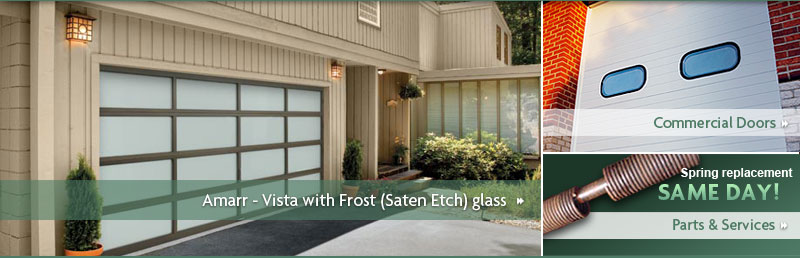The image appears to be a screenshot from a door-related website, featuring a split layout. The larger section, occupying approximately 75% of the rectangular box, showcases an image of a residential garage door labeled "Amar-Vista with Frost (satin etch) glass." This section is overlaid with a light, transparent green highlight and includes a forward play button.

To the right, in the smaller 25% segment, there is an image depicting a commercial door on a building, which features two windows. This section is highlighted with a transparent white bar, with the text "Commercial Doors" prominently displayed in green. Below this, there is additional text offering "Spring Replacement" and "Same Day Parts and Services," which also features an illustration of a roll-up door component in bronze.